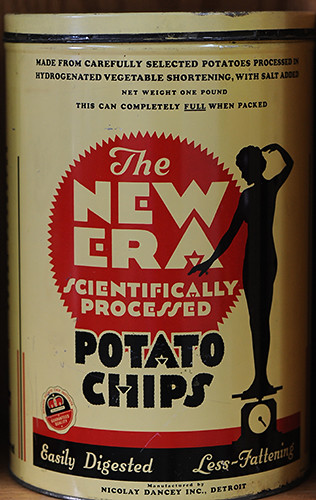The image depicts a vintage, beige tin can, approximately twice as tall as it is wide, filling almost the entire frame with a medium brown border around it. The can, which likely dates back to the 1960s or 1970s, features black text at the top that reads: "Made from carefully selected potatoes, produced by hydrogenated vegetable shortening with salt. Net weight one pound. This can be completely full when packed." In the center, a red circle with jagged edges has white lettering that says "the new era scientifically processed," and below that, in black lettering, it states "potato chips." Additionally, there is a black silhouette of a woman standing on a scale as part of the logo, and at the bottom of the can, it reads: "easily digested, less fattening."